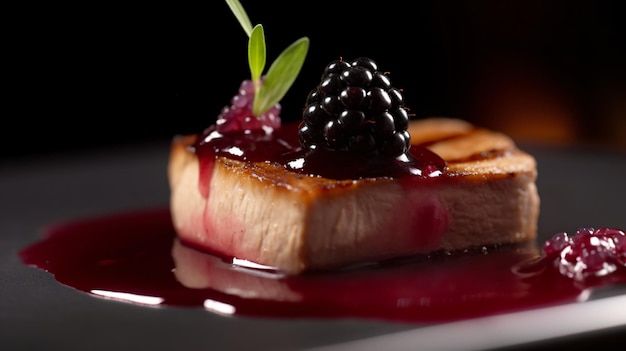This close-up angled photograph displays a meticulously grilled square piece of salmon, prominently featuring distinct left-to-right sear marks. The salmon hosts a single, plump blackberry on its top, with a raspberry glaze artfully dripping down its sides. Accompanying this is a dollop of purplish caviar nestled in the top left corner, adorned with two delicate sprigs of lemongrass at the center. The presentation rests on a gray plate that is itself encircled by a glossy pool of blackberry glaze, creating a visual contrast. The dish is captured in sharp focus against an out-of-focus, black backdrop, emphasizing the gourmet elegance and intricate details of the food.